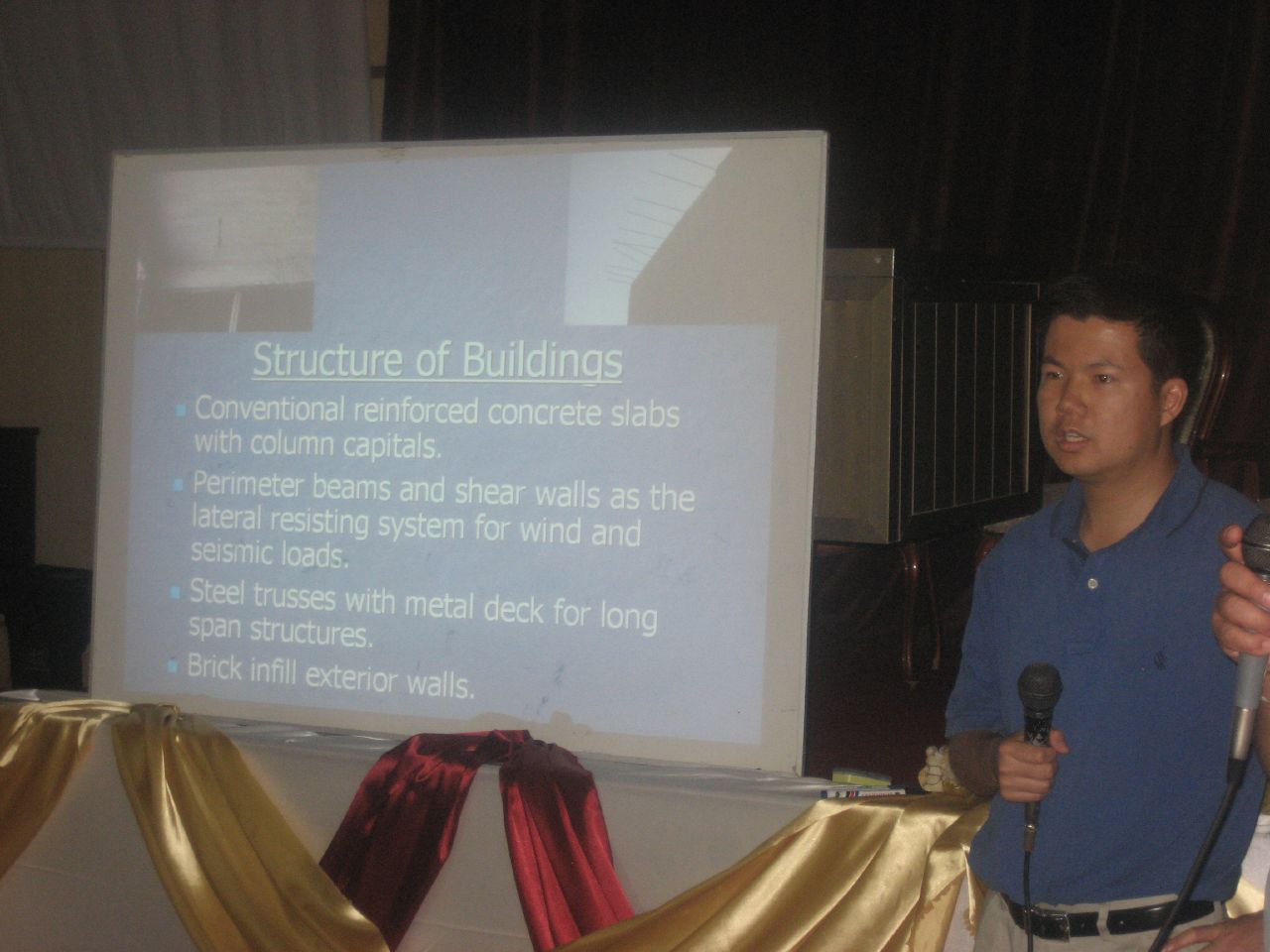The image depicts a man, who appears to be of Asian descent and has dark, short hair, standing on a stage or in a conference room. He is positioned towards the bottom right of the image, facing forward and slightly to the left, wearing a bluish-gray button-down shirt tucked into light gray trousers with a black belt. The man holds a black microphone in his right hand, which is held chest-high. 

To his left, centrally located in the image, is a large screen or poster displayed on a white table draped with a tablecloth adorned with gold and maroon ribbons. The screen features the headline "Structure of Buildings" underlined prominently. Below this headline, there are four blue bullet points, each followed by white text describing various structural elements: "Conventional reinforced concrete slabs with column capitals," "Perimeter beams and shear walls as the lateral resistance system for wind and seismic loads," "Steel trusses with metal deck for long-span structures," and "Brick infill exterior walls."

In the background, a dark wall suggests the setting is indoors, likely a presentation or lecture in a conference room. The presence of a second microphone held by an unseen person suggests the man is addressing an audience. The overall scene is meticulously decorated and well-organized, emphasizing the formal nature of the event.